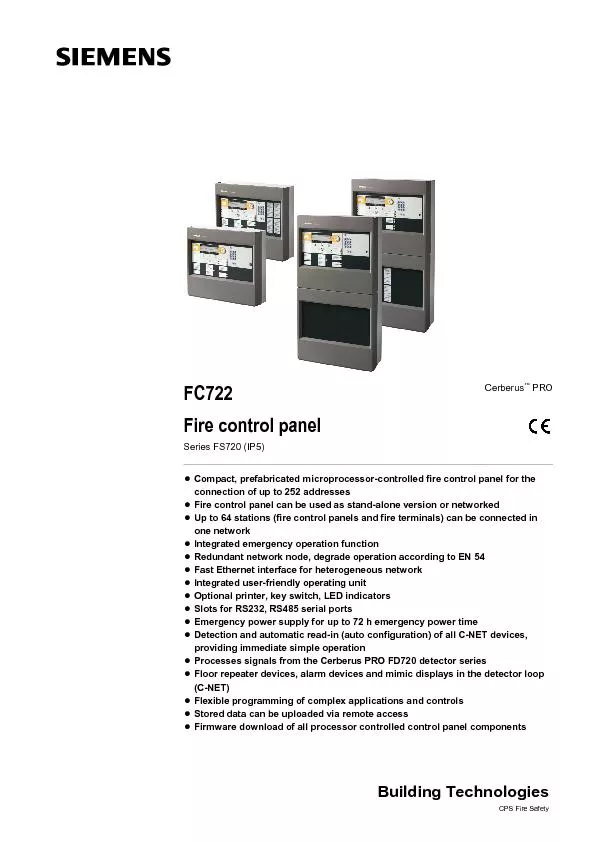The advertisement showcases Siemens Fire Control Panel FC722 from the FS720 series, emphasizing its advanced fire safety technology. The ad prominently features four images of the control panels, each equipped with various knobs, switches, and microprocessor components. At the top left corner, the Siemens logo is displayed boldly in black capital letters. Below the images, the model number "FC722" is also highlighted in black capital letters, followed by the detailed product description "Fire Control Panel" in mixed capitals and lowercase letters.

Additional information includes "Sirius FS720 (IP5)" in smaller print beneath the main description. On the right side of the page, the Cerberus Pro CE features are elaborated, listing key characteristics such as the ability to connect up to 252 addresses, network compatibility for up to 64 stations, and integration capabilities with emergency operation functions. The panels support fast Ethernet interfaces, RS-232, and RS-485 serial ports, and offer a robust emergency power supply lasting up to 72 hours. The design incorporates user-friendly elements including LED indicators, optional printers, key switches, and flexible application programming for complex controls. The panels are compatible with the CERBIUS PRO-FD720 detector series, along with various alarm and mimic display devices, enabling seamless and efficient fire safety management.

The advertisement concludes with "building technology" and emphasizes the product's benefits for fire safety under CPS Fire Safety, demonstrating Siemens’ comprehensive approach to modern fire control solutions.